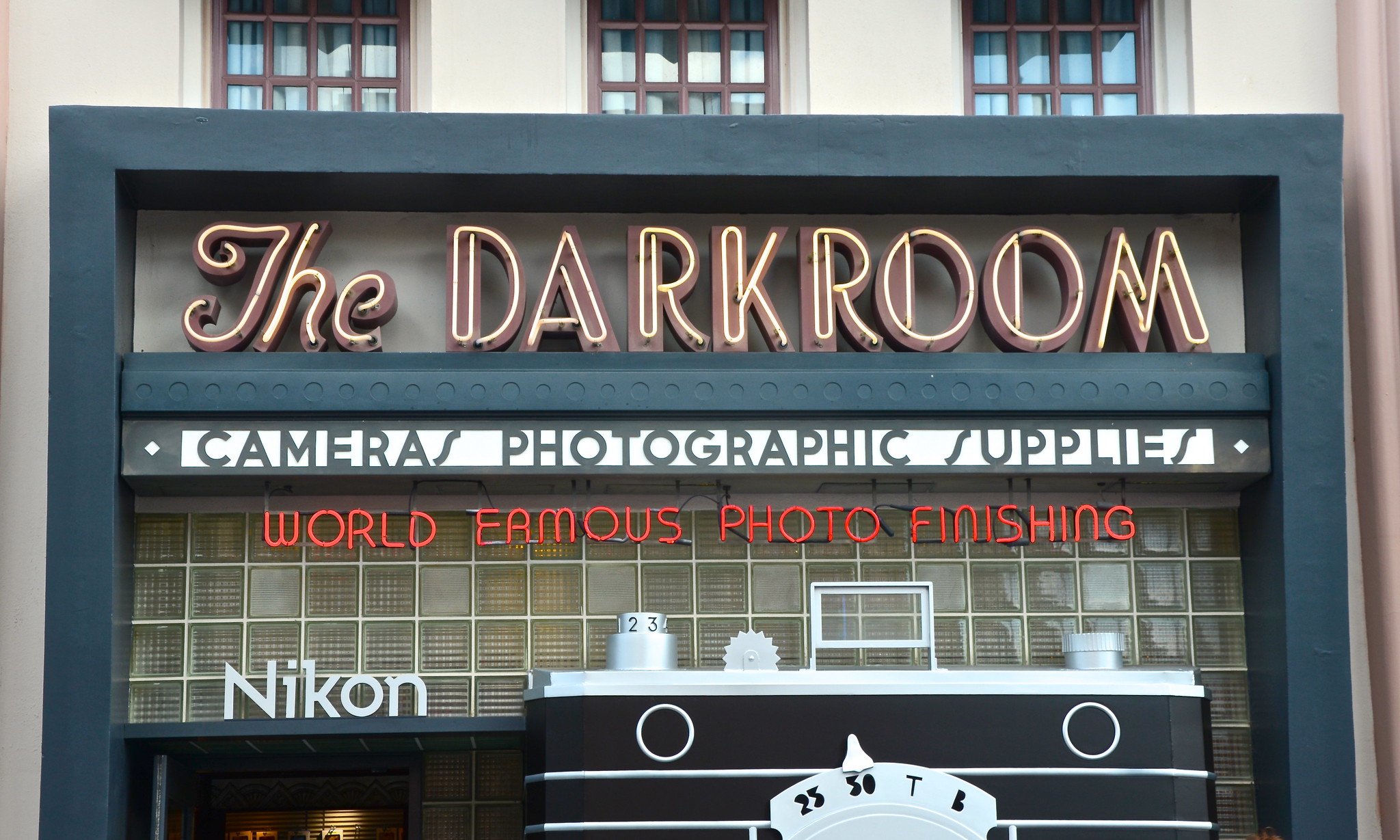This photograph captures the exterior of a white camera store situated on the ground floor of a two-story building, possibly an apartment complex, identifiable by its three second-story windows with blinds. The tan stucco facade gives way to a prominent sign framed by what appears to be a dark bluish-black metal bar. The sign features "THE DARK ROOM" in large, theatrical 1940s-style black lettering, with "THE" scripted in a cursive font above it. Directly beneath is another sign that reads "CAMERAS PHOTOGRAPHIC SUPPLIES." Further down, a neon sign in red lettering proclaims "WORLD-FAMOUS PHOTO FINISHING," likely glowing in the dark. To the left of this neon sign is the store's entrance, marked by the "NIKON" logo in white letters above the door. Adjacent to the door, on the building's exterior, is a large, sculptural representation of an old-fashioned camera, likely constructed from metal and concrete, adding an artistic touch to the storefront. The overall ambiance of the scene suggests it was taken on an overcast day, as the lighting appears subdued.